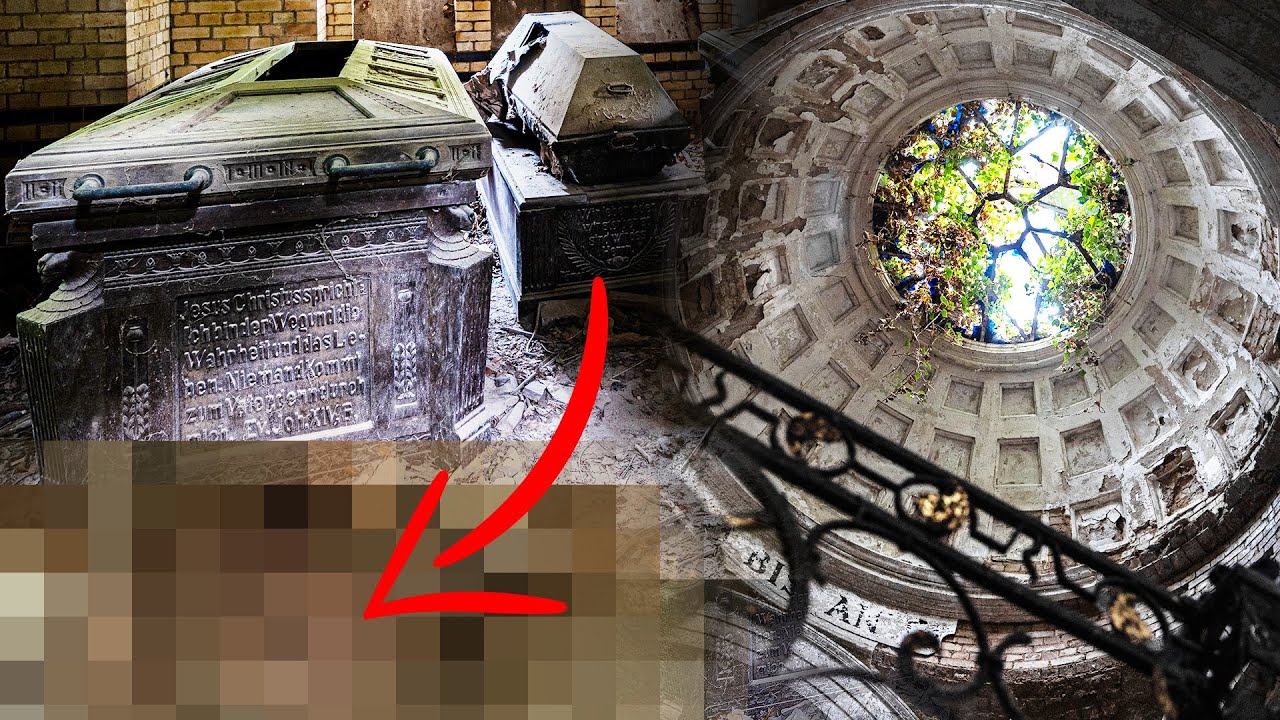The image captures the interior of a cylindrical atrium within a building, characterized by window-shaped rectangles carved into the stone walls and ascending in a cylindrical pattern. The focal point is a massive skylight at the top, which floods the space with natural sunlight, revealing glimpses of trees outside. On the left side, there is a closed coffin or sarcophagus adorned with inscriptions. A red arrow points from the inscriptions to the lower left corner of the image, which is heavily pixelated and blurry, reminiscent of TV censorship. The right side features a dome-shaped skylight that brings in sunlight, with leaves or trees visible through the glass, adding to the grandeur of the cylindrical, cathedral-like architecture.